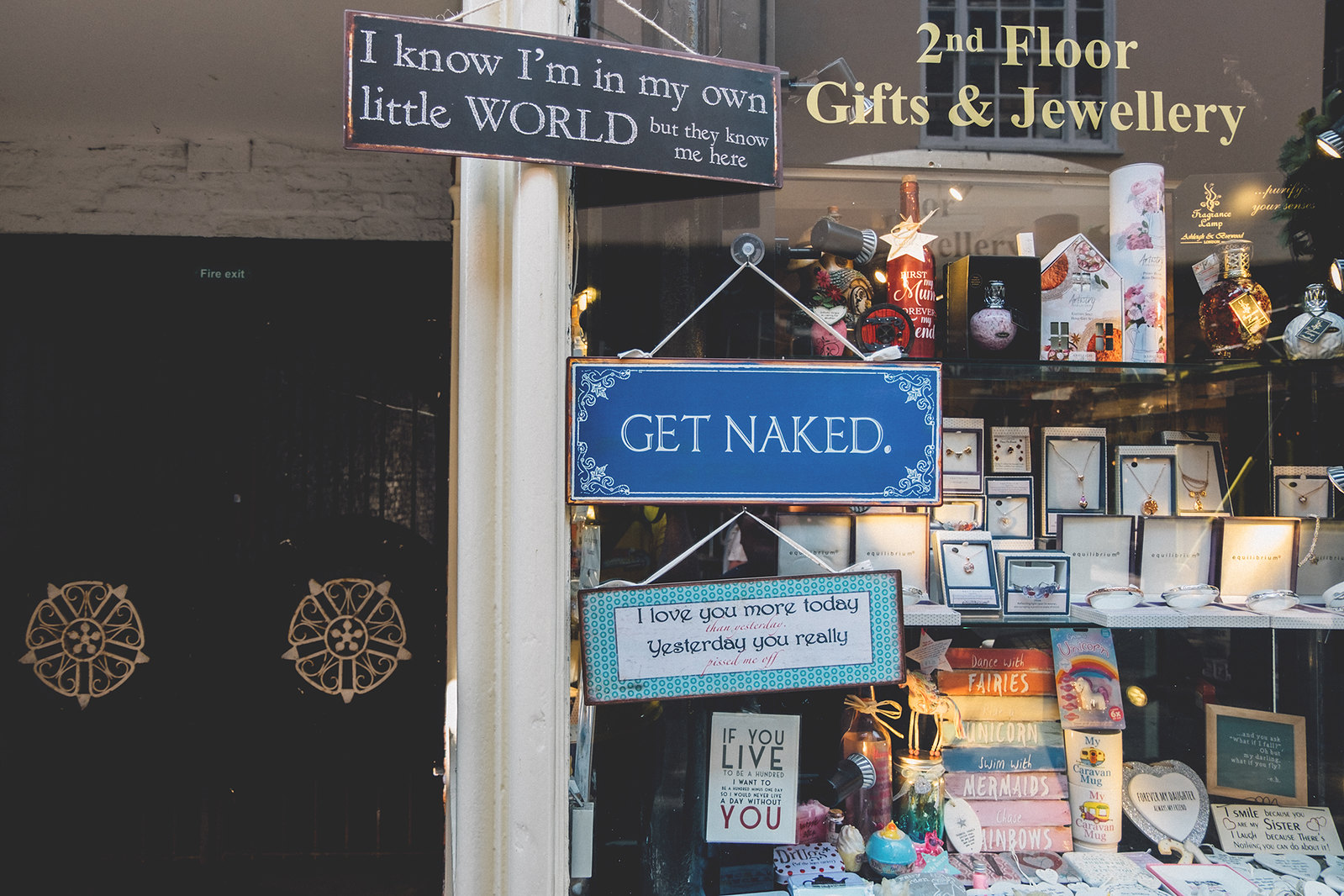This detailed, color photograph captures an exterior scene of a storefront in a shopping district, oriented in landscape. The left-hand side features a vertical white trim border running from top to bottom, adjacent to dark gray and black walls. A prominent sign at the top of this border reads, "I know I'm in my own little world, but they know me here." Beside it, the storefront is visible through a large glass window. The top of the window features yellow lettering that says, "Second Floor Gifts and Jewelry." Hanging from the window on the left-hand side are three signs with playful messages: "Get Naked," "I love you more today than yesterday. Yesterday, you really pissed me off," and "If you live to be a hundred, I want to never live a day without you."

Inside the window, three shelves display a variety of items. The top shelf holds potpourri and fragrance items, the middle shelf showcases boxed jewelry, and the bottom shelf is filled with keepsakes and knickknacks. There are also mugs and other small signs with whimsical phrases like "Dance with fairies," "Swim with mermaids," and "Chase rainbows." To the far left are two black doors with ornate gold handles. The photograph captures the detailed and eclectic nature of the shop’s offerings, exemplifying a quaint, inviting atmosphere.